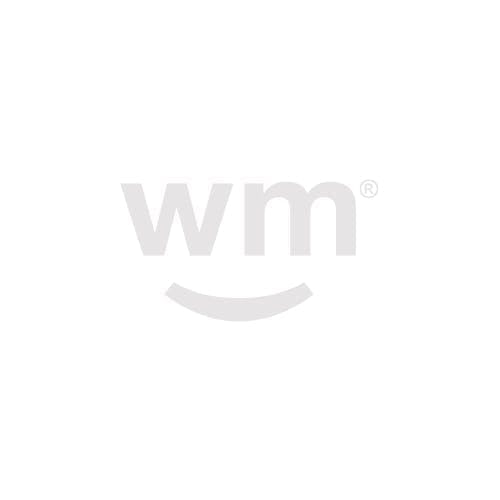In the center of a predominantly white background, there is a minimalist and very light gray (almost white) company logo. The logo features the lowercase letters "w" and "m," followed by a registered trademark symbol (®). Beneath these letters is a subtle swoosh-shaped line, reminiscent of a small smile, extending from the left under the "w" to just below the middle of the "m." The entire logo is centralized on the white background, giving an impression of simplicity and modernity, potentially suitable for a technology-related company.